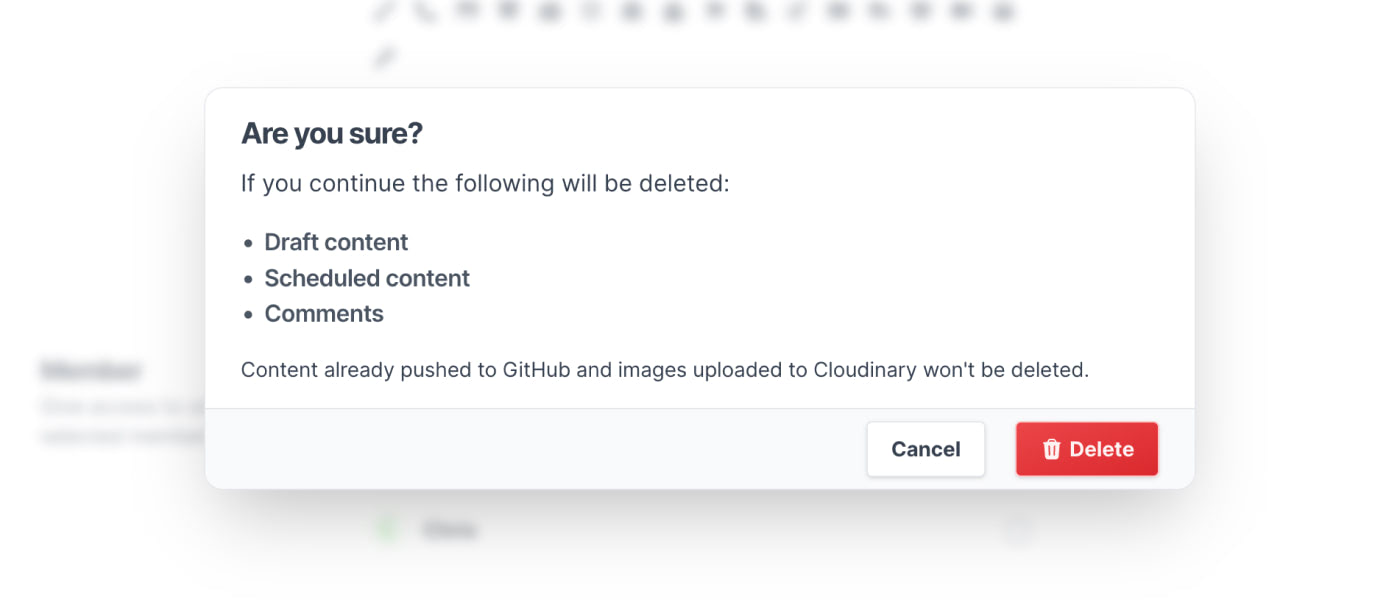The image depicts a file deletion popup on the GitHub website, set against a white background. Dominating the center of the screen is a large white box. At the top left corner of this box, the words "Are you sure" stand out in bold black letters. Directly below this heading is additional text that states, "If you continue, the following will be deleted," followed by a bullet-point list detailing three items: draft content, scheduled content, and comments.

Further down, a smaller black font informs users that "content already pushed to GitHub and images uploaded to Cloudinary won't be deleted." In the bottom right corner of the popup, there are two interactive buttons. The left button, a white box with the word "Cancel" in bold black letters, offers an option to abort the action. To its right, a red box with the word "Delete" in white letters serves as the confirmation button for deleting the specified items.

The background behind the popup is slightly blurred, revealing a faint image of what appears to be a GitHub page. Icons are visible along the top center of this background, and on the bottom right, a category header in bold black letters is noticeable, followed by smaller black text detailing the category information.